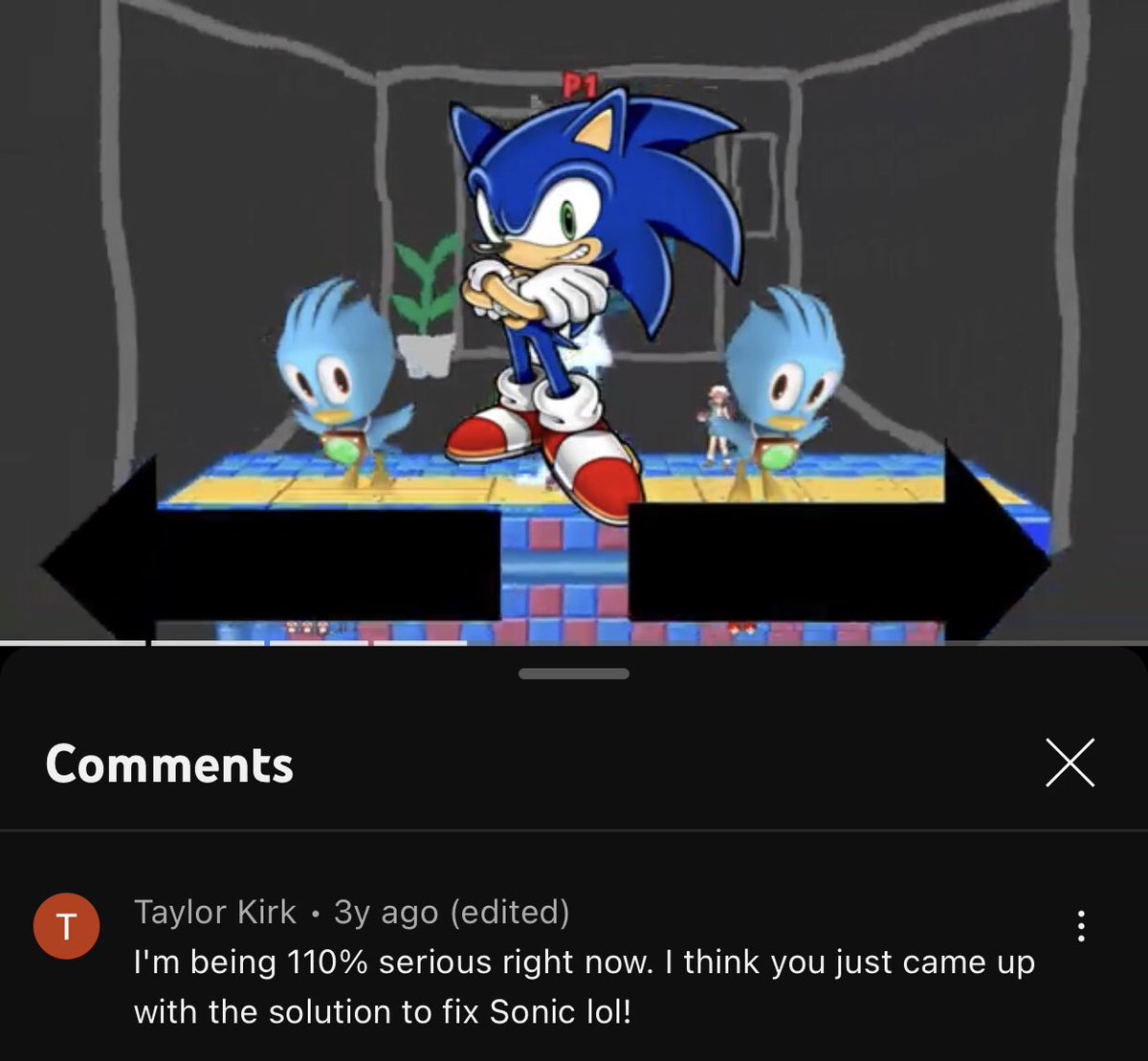In the screenshot, a distinctive scene features Sonic the Hedgehog standing inside a cozy house. Flanking Sonic are two animated birds—one perched on his left and the other on his right. Above Sonic's face, a 'P1' marker is prominently displayed. Below Sonic, there are two black arrows: one points to the right, and the other points to the left, possibly suggesting movement options or choices.

Overlaying the image, there is a dialogue box containing a comment highlighted by a red circle with a white 'T' icon, indicating an interaction by a user named Taylor Kirk. The comment reads: "I'm being 110% serious right now. I think you just came up with the solution to fix this. Sonic, L-O-L!" This comment has been edited, as indicated by the word 'edited' in parentheses. Near the top-right corner of the comment box, there are three vertical dots, likely for additional options such as editing or deleting the comment. Lastly, an 'X' icon is visible, possibly for closing the comment box.